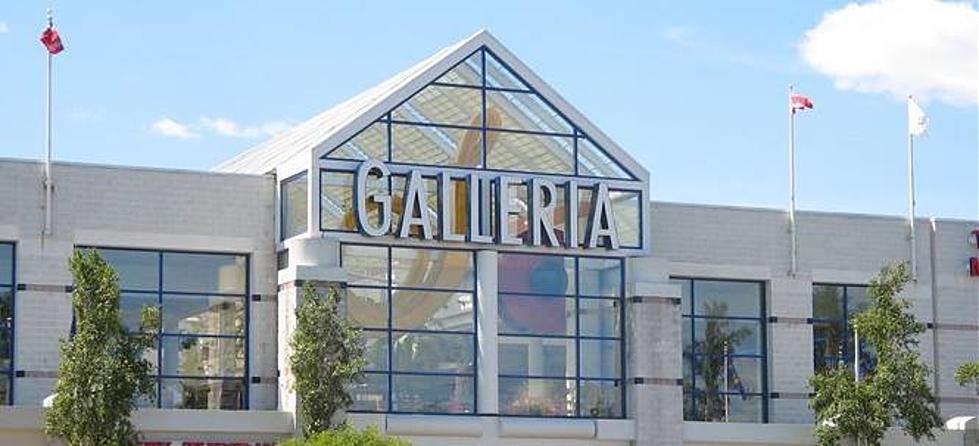The image is a full-color photograph taken outdoors on a mostly sunny day with a clear blue sky and a few white, puffy clouds in the upper right corner. The photograph features a modern white building with a lot of glass windows and a distinctive glass gabled roof in the center. Boldly displayed on the front of the building is a sign reading "Galeria." In front of the building, there are four green shrubs, adding a touch of greenery to the scene. Three flagpoles are visible, one on the far left and two on the right, displaying flags in red, white, and possibly other colors, signifying various countries. The architectural style of the building is contemporary, and it is concrete with extensive use of glass, including a decorative glass roof over a triangulated area. The photograph captures the building slightly off-center, with lush green trees around, suggesting late spring, summer, or early fall. This setting might indicate that the place could be a shopping mall, an art gallery, or a museum.